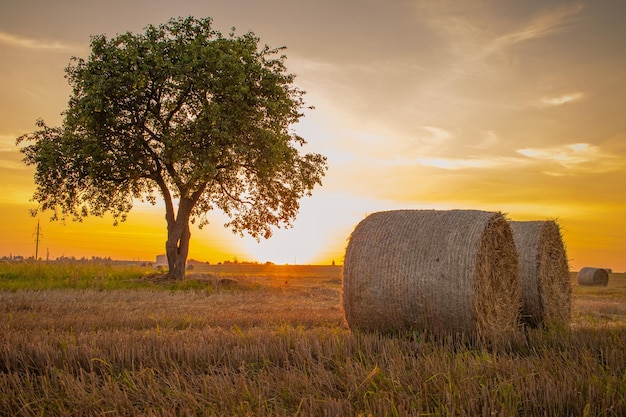This image, likely a painting, depicts a serene agricultural setting at sunrise or sunset. Dominating the foreground are two large, rolled hay bales positioned side-by-side towards the middle right. A third hay bale is visible in the distance. A solitary tree with green leaves and multiple trunks stands in the background, slightly left of center, reaching towards the top of the image. The landscape stretches into a vast, recently harvested field which may once have been filled with wheat. The horizon line extends from the left to the right about midway down the image. The sky displays a captivating gradient, transitioning from a golden yellow at the horizon, where the sun rises or sets, to a grayish-blue towards the top. The scene is bathed in warm hues of white, yellow, beige, and orange, contrasted by the greens of the tree and field, creating a peaceful and pastoral atmosphere.